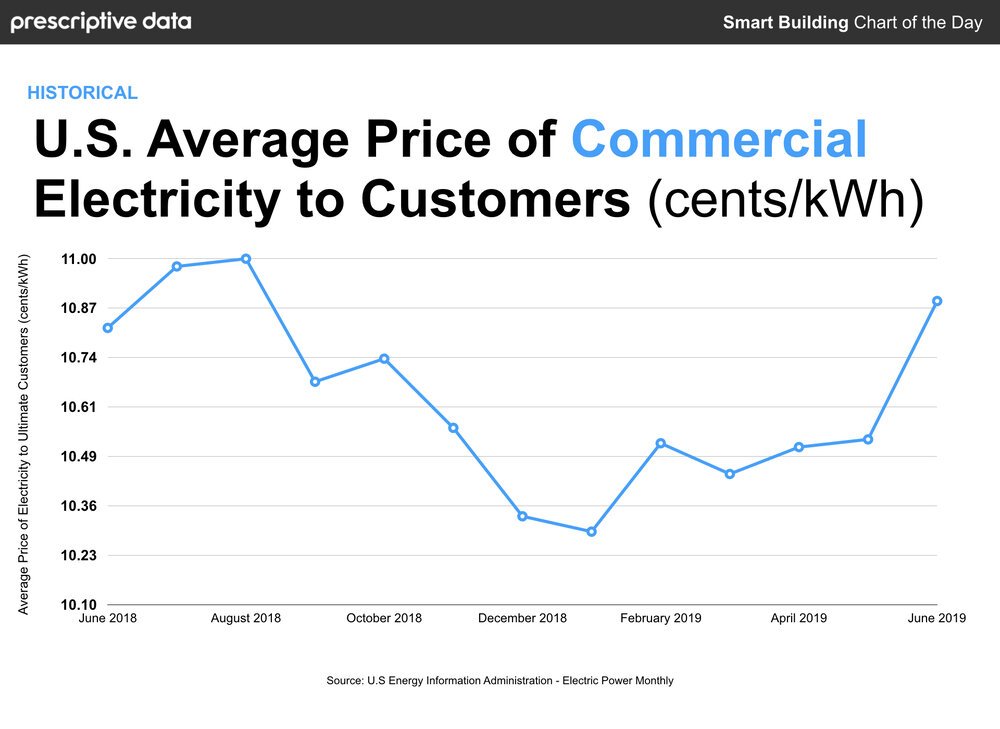The image is of a scientific chart that appears to be something featured in a magazine or scientific journal, focusing on the U.S. average price of electricity for commercial customers. The chart is titled "Prescriptive Data" in white text on a large dark gray rectangle at the top, with the phrase "Smart Building Chart of the Day" to the right. Below this title, in blue text, is the word "Historical." In large, black text is "U.S. Average Price of Commercial" with "Commercial" in blue. This is followed by "Electricity to Customers (cents/kWh)" in black text.

The chart prominently features a blue line graph with dots, illustrating the changes in electricity prices for commercial customers over time. It spans from June 2015 to June 2019, tracking the monthly fluctuations in price. Key months such as August 2018, October 2018, December 2018, February 2019, April 2019, and June 2019 are marked. The numerical range on the graph's Y-axis starts at 11 and goes down to 10.10, showcasing detailed data points on electricity pricing, aimed at aiding builders in constructing smart buildings.